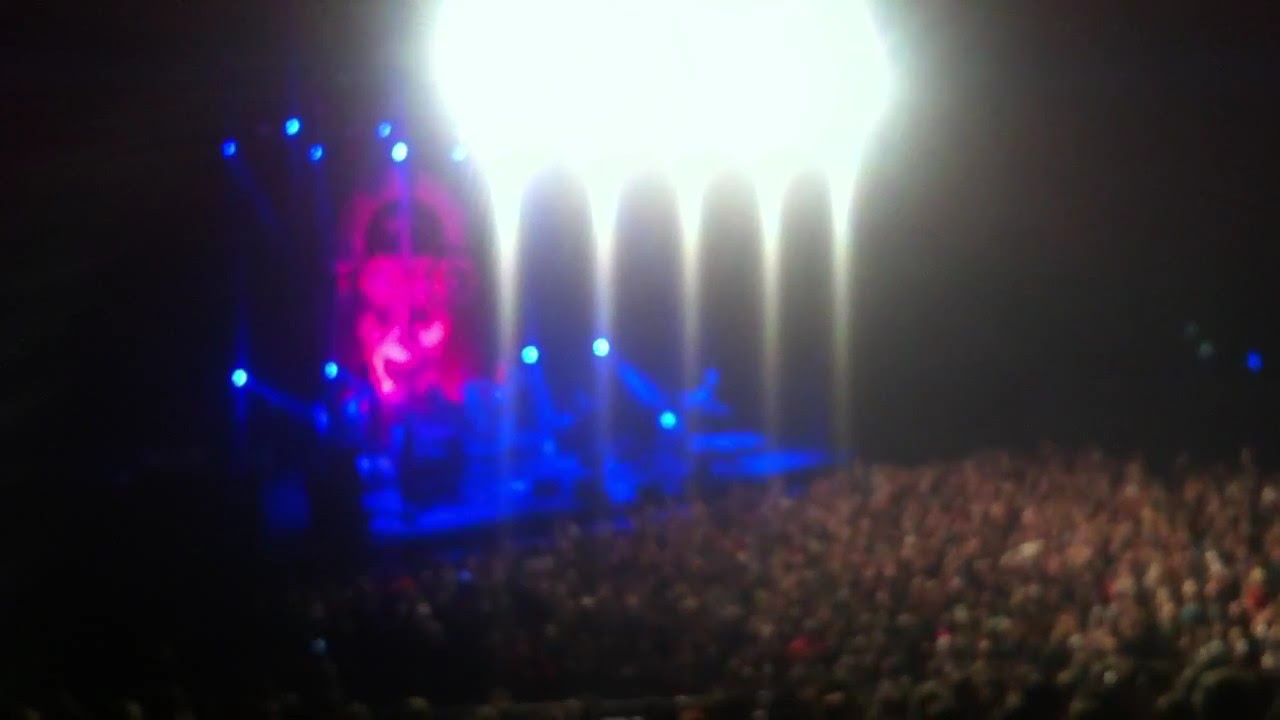In this image of a concert, the venue is densely packed with a vibrant crowd occupying the lower right section, stretching from the left corner to the midpoint of the right side. The stage, located on the upper left, is enveloped in an intense, saturated blue light with several white lights interspersed around it. The bluish hue casts an ethereal glow, creating a somewhat surreal atmosphere. Dominating the background is a smiling face projected in pink hues, although the poor image quality makes it challenging to identify the person or activity on stage. At the very top, five intensely bright lights beam downwards, their brilliance almost obscuring their sources, resembling radiant rays of the sun. Despite the blurred and out-of-focus nature of the photograph, the energy and scale of the concert are palpably immense, suggesting a lively and heavily attended event.